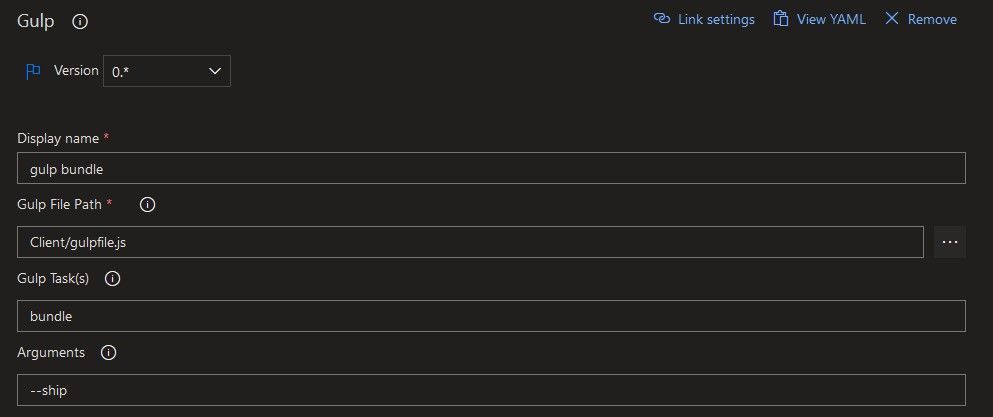### Screenshot of Gulp Configuration Interface for File Sharing or Programming

This landscape-oriented screenshot showcases a user interface from a file sharing or programming app, set against a sleek black background. 

**Header Section:**
- At the top, in white text, is the label "Gulp," adjacent to an information icon represented by a white bubble with an eye inside it.
- To the right of this, there are three blue buttons:
  - **Link Settings** - with an accompanying icon.
  - **View YAML** - also with an icon for visibility of the file format.
  - **Remove** - featuring an icon for function execution.

**Version Dropdown:**
- Below the "Gulp" label on the left, a blue flag icon is followed by the text **Version**. 
- There is a dropdown box with a white border containing **0*** (zero asterisk) and a down caret, indicating the selection and availability of more versions.

**Configuration Fields:**
- The first field header is **Display Name** marked with a red asterisk (indicating a mandatory field), pre-filled with **Gulp Bundle**.
- Below this is the **Gulp File Path** field, accompanied by an information icon. Inside the text box, it reads **client/gulpfile.js** with an ellipsis (three-dot) icon for file browsing functionality.
- Next is the **Gulp Tasks** field, which contains the entry **bundle**.
- Lastly, the **Arguments** field pre-filled with **--ship** is displayed.

Each text box features a white border and white text, enhancing readability against the dark theme.